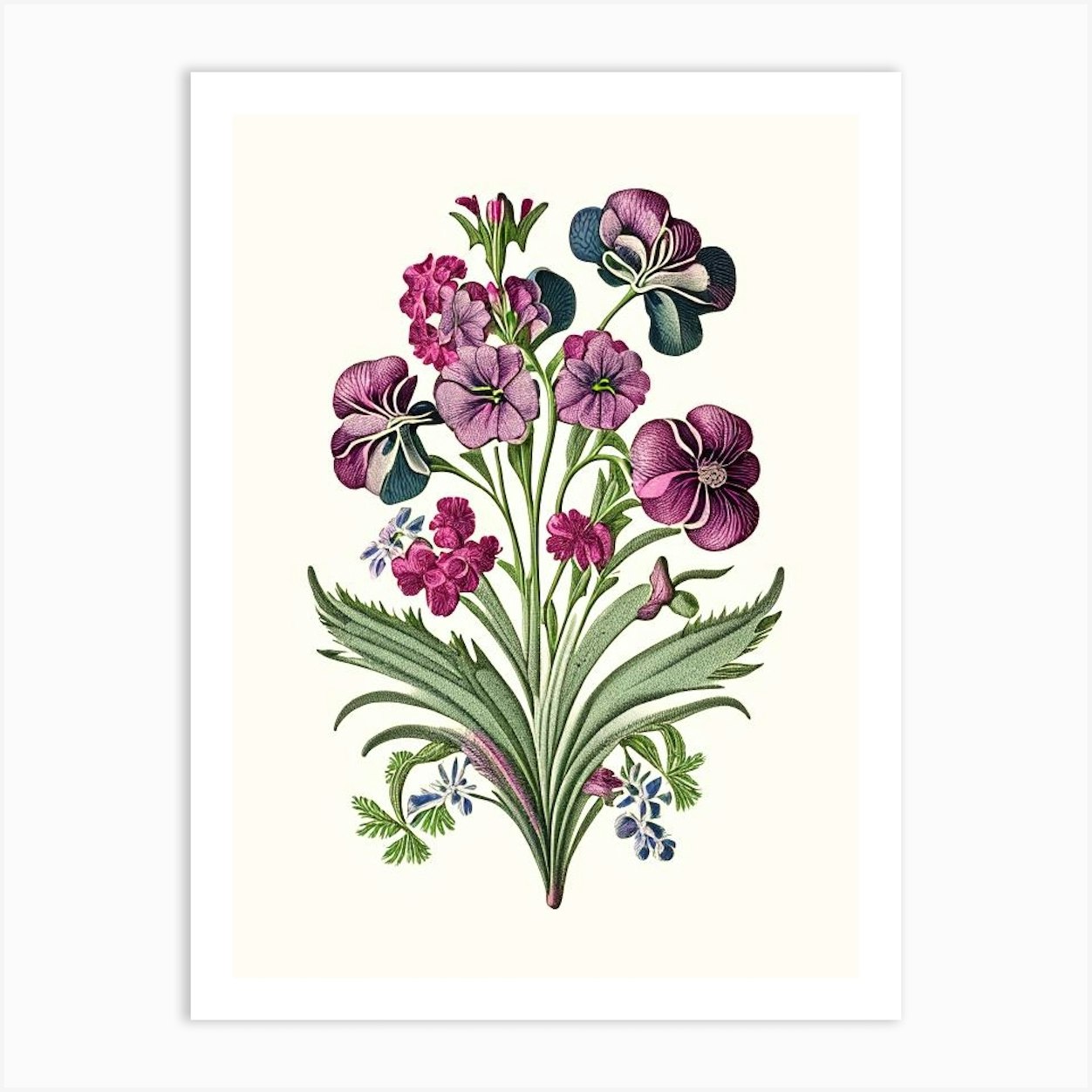The image is a hand-drawn illustration of a flower bouquet, set against an ivory background with a white border. The bouquet features green stems that rise from the bottom, leading to a variety of flowers in purplish and pink hues, some with blue accents. The flowers vary in size and shape, with most of them open but a few still closed. At the bottom of the bouquet, there are two large green leaves accompanied by smaller leaves of different sizes and shapes, adding to the intricate detail of the artwork. The flowers and leaves are carefully depicted on a textured cardstock paper, highlighting the artist's attention to realism and detail.